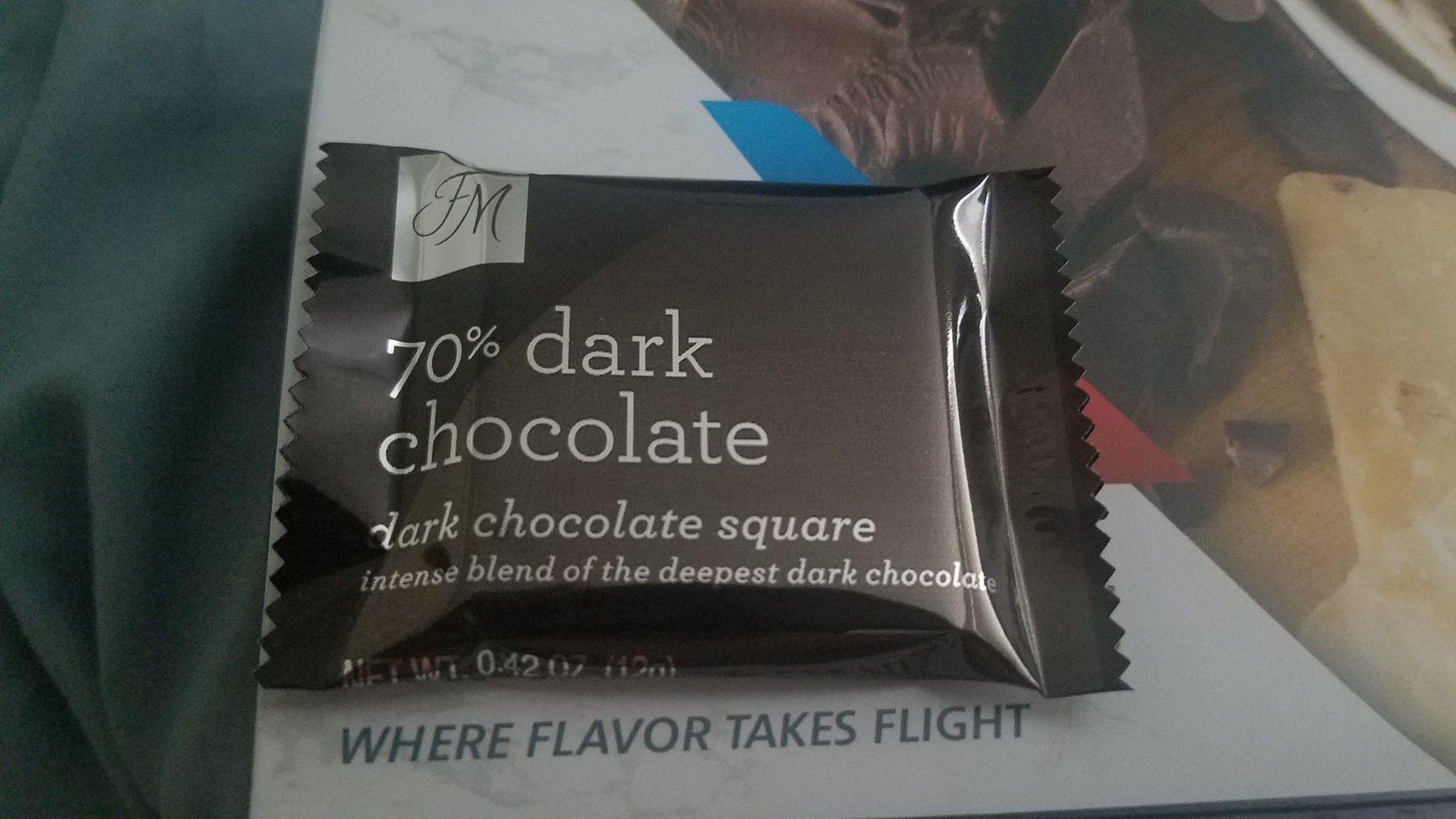The image showcases a photorealistic, close-up view of a piece of dark chocolate in its wrapper. The wrapper is a shiny dark brown, made of paper plastic, and features serrated edges. In the upper left corner of the package, there is a silver square with the initials "FM" in black font. The central part of the wrapper prominently displays the text "70% Dark Chocolate" in white font, followed by "Dark Chocolate Square," and the description, "Intense blend of the deepest, darkest chocolate." The net weight of the product is 0.42 ounces. The chocolate is placed on a piece of paper, which appears to include images of chocolate, possibly scanned onto it. At the bottom of this paper, the phrase "Where Flavor Takes Flight" can be seen, along with other designs featuring brown, blue, and red colors. The piece of paper rests on a darker green fabric that is wrinkled, partially visible to the left, and hints at an airport flyer or similar setting. A gleam of light is noticeable on the chocolate packaging, enhancing its shiny appearance.